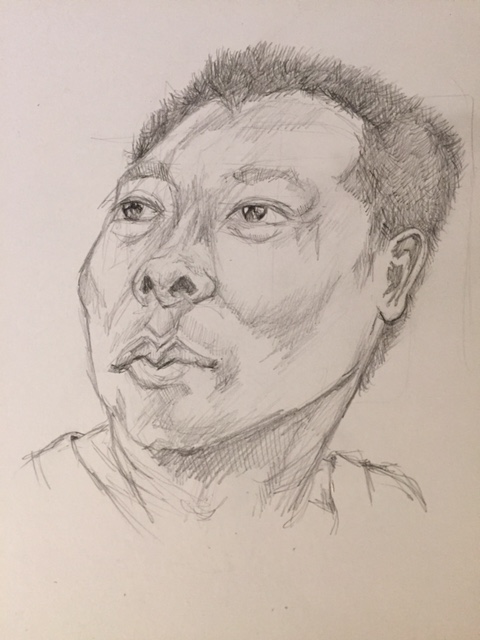This vertically oriented color sketch captures a detailed portrait of a man rendered in pencil. The subject, an African-American man, is depicted from the neck up, with only a sliver of his neck and shoulders visible. His head is tilted back as he gazes upward to the top left corner of the image. The man has short, cropped hair, styled in a slight V-shape at the forehead. Distinctive features include his well-defined cheekbones, strong nose, and prominent mouth. His left ear is visible, and his eyes, accentuated with light and dark shading, give a sense of depth and emotion. The overall shading in the portrait uses a range of gray tones, contributing to the lifelike quality of the drawing. This detailed sketch is executed on slightly off-white paper, further enhancing its textured, realistic appearance.